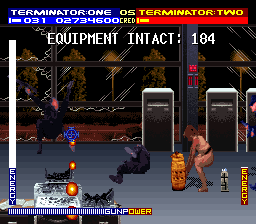The image depicts a screen from a computer game, likely during an intense action sequence. At the top of the screen, in blue text, it reads "Terminator 1" and "OS," while on the right, it says "Terminator 2." Below that, in a lighter blue text, is the sequence "031 0273-4600," followed by "Equipment Intact: 184" in bold capital letters. 

The background features a combination of black and gray tones, with the scene seemingly taking place outdoors on a rainy night, indicated by diagonal white lines resembling rain. There are greenish-brown trees and yellow diamond-shaped street signs visible through large, rectangular, black-framed windows.

In the center of the scene, a female character is depicted in a squatting position, appearing to lift an object. In front of her, a male character in black clothing with a red and blue mask is in mid-fall, with his left leg up and his right arm raised, suggesting he was shot. Another character, also in black and possibly a ninja, is seen lying on the ground with one leg up and his body falling backward.

Additional text on the screen includes labels such as "energy" on the bottom left, "gunpower" in the middle bottom, and "energy" on the bottom right. The color palette of the scene includes red, blue, yellow, orange, tan, brown, gray, black, and white, providing a visually dynamic and detailed environment.